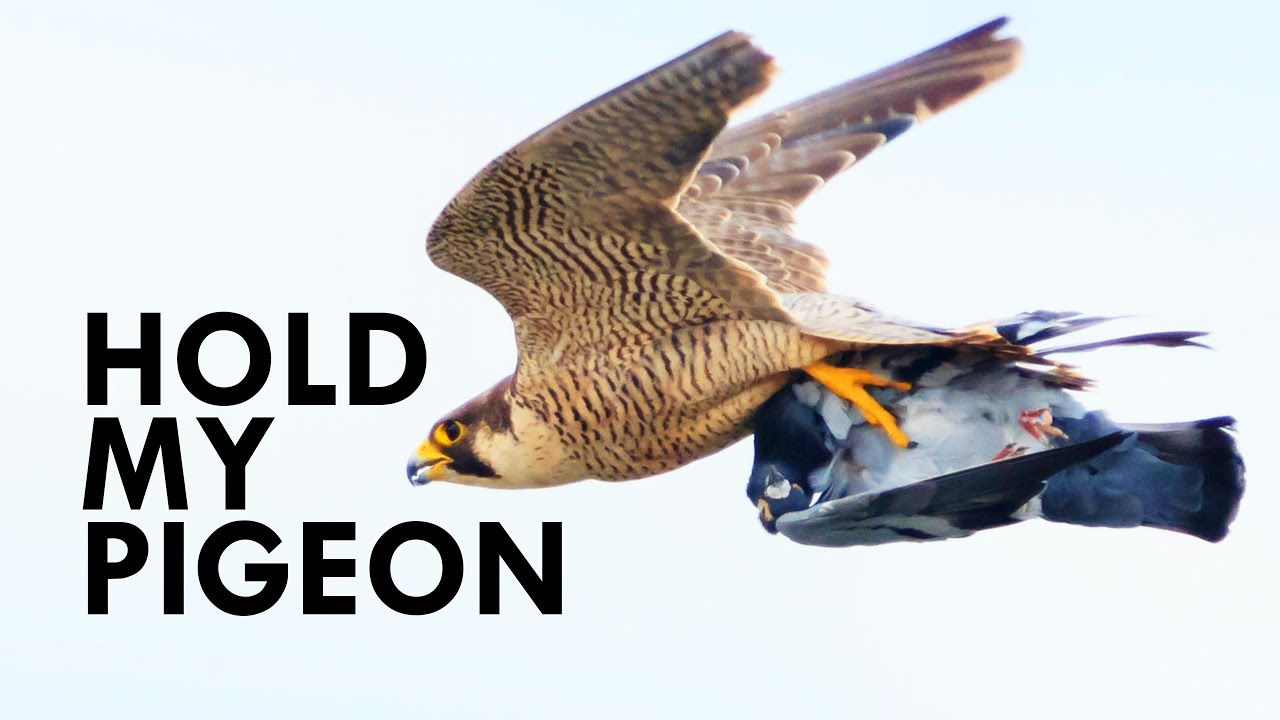In the center and right of the image, a light brown bird with dark brown stripes is depicted mid-flight, its wings spread wide. The bird features striking details, including a yellow beak with blue accents, black eyes, and brilliantly bright yellow claws. Clutched in its claws is a pigeon with dark blue feathers, a light blue belly, and tiny pink feet, suggesting it is the bird's prey. Above the scene, bold black text reads "hold my pigeon," with the pigeon's head aligning between the letters. The background is a pale blue, reminiscent of the sky, tying the whole image into a picturesque and dramatic capture of nature.